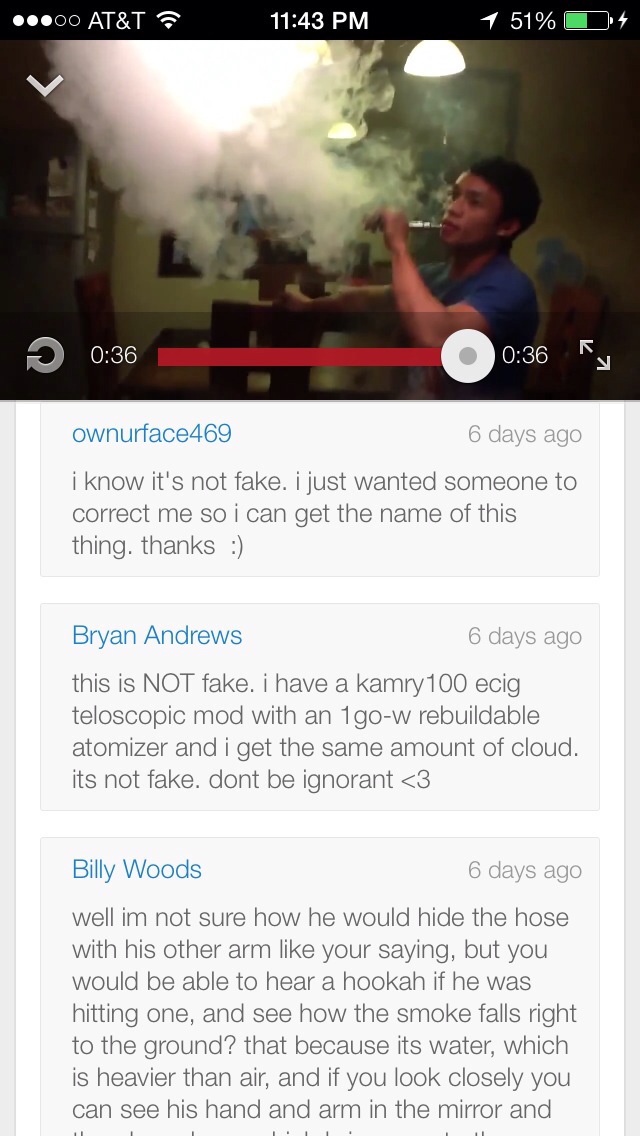This is a screenshot of a 36-second video clip showing a man vaping, expelling a huge white cloud of smoke. At the top, the smartphone interface displays details such as AT&T service, a Wi-Fi connection, the time 11:43 PM, and 51% battery life. In the video, the man is seated in a room, blowing a large amount of smoke. Below the video, there's a white background with light gray boxes containing comments from three different users. The first comment, by ownerface469 in blue, posted six days ago, reads, "I know it's not fake I just wanted someone to correct me so I can get the name of this thing, thanks." The second comment from Brian Andrews, also posted six days ago, states, "This is not fake. I have a Camry 100 ESIG telescopic mod with a 1GOW rebuildable atomizer and I get the same amount of cloud. It's not fake, don't be ignorant." The final comment by Billy Woods, posted six days ago, says, "Well, I'm not sure how he would hide the hose with his other arm like you're saying, but you would be able to hear a hookah if he was hitting one, and see how the smoke falls right to the ground? That's because it's water, which is heavier than air. If you look closely, you can see his hand and arm in the mirror..." which then gets cut off.